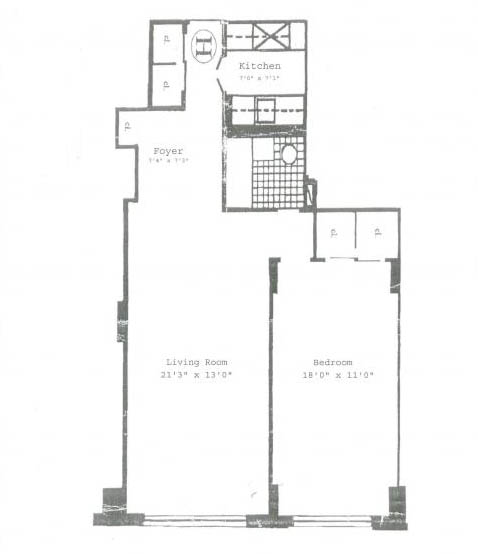This is a meticulously detailed drawing with a white background, depicting the layout of someone's house. 

Starting at the bottom left corner, there's a bedroom labeled "110." This bedroom features two small closets. Adjoining this bedroom to the right is a substantially larger room denoted as the living room, with dimensions of 213 by 130. These two rooms comprise the bottom section of the house.

Moving upward, there is a foyer situated centrally. Positioned above the foyer is a marked area with an "H" enclosed in a circle. Flanking the foyer are two rooms labeled "CL" on both sides.

Directly above the living room is an area with a distinctively drawn tile flooring pattern, including a circle and a square. This serves as a transitional space leading to the kitchen above. The kitchen's dimensions are not legible, but it connects to two small adjacent rooms.

Overall, the drawing intricately details various rooms and features within a house, providing a clear and comprehensive floor plan.